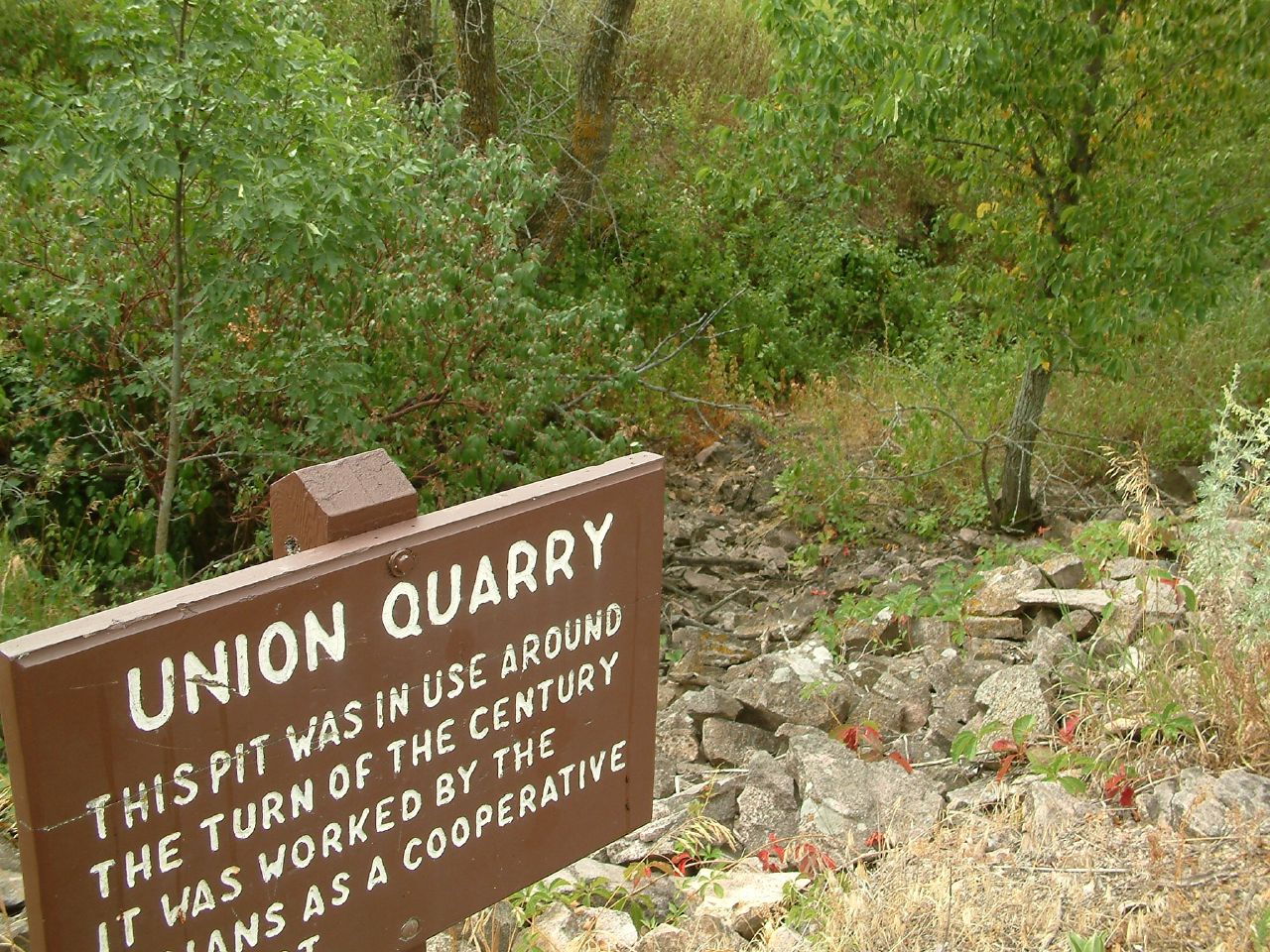This daytime photograph captures a historic, outdoor scene looking down a rocky hillside into a valley filled with trees, bushes, and various vegetation reclaiming the area. In the foreground at the bottom left, there is a weathered wooden sign angled from the lower left to the upper right, bearing white, partially visible text. The sign reads "Union Quarry" at the top, followed by "This pit was in use around the turn of the century. It was worked by [illegible] as a cooperative," with the final line cropped out. The image features an array of earthy colors, including browns, grays, tans, greens, and hints of orange and yellow. The lower right corner shows brush and ivy growing between large gray rocks, while the top half of the image is dominated by shrubs nestled in the valley below, emphasizing nature's reclamation of this historical site.